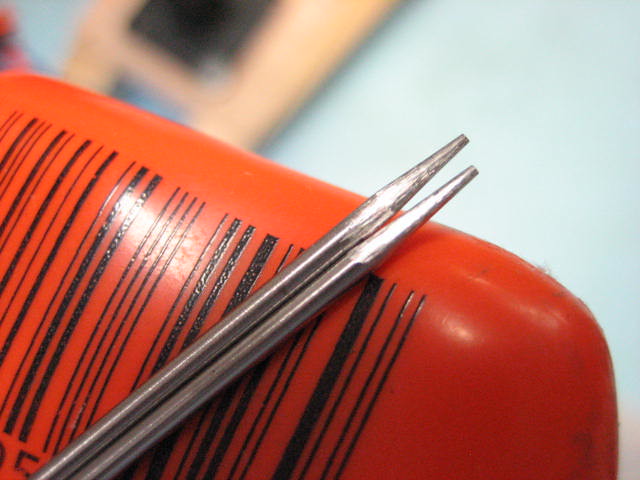The image depicts two slender, silver metal rods with pointed tips, appearing similar to needles or probes. These rods are positioned diagonally from the bottom left to the top right of the image at an approximate 45-degree angle. They lie atop a red object that features black barcodes, with the number '5' visible beneath one of the barcodes. The red object itself is oriented in the opposite direction, extending from the top left to the bottom right. The background is a pastel light blue with a blurred square shape featuring a section of a black square. The focus of the image is sharply on the two metal rods and the red object, highlighting their metallic sheen and barcode details against the soft, indistinct backdrop.